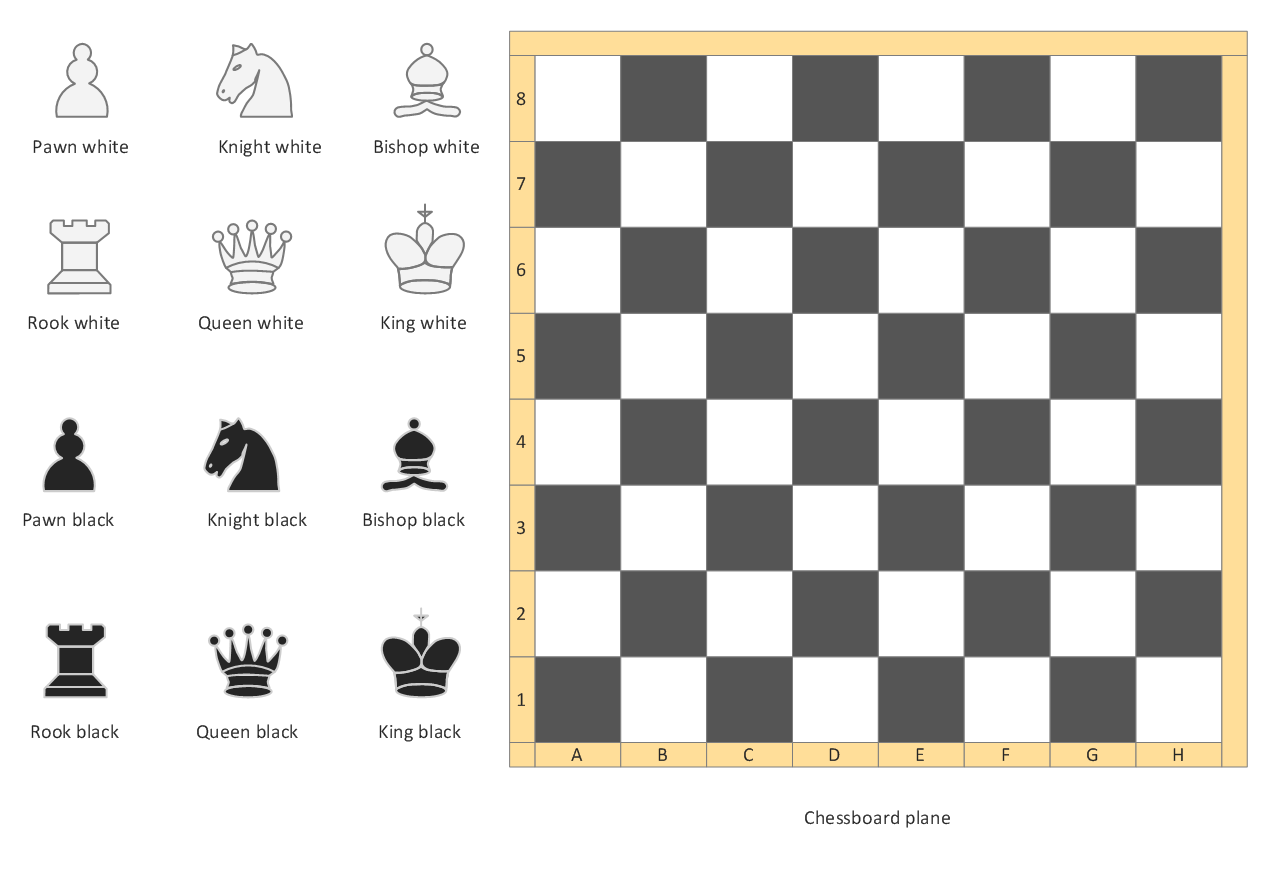This image is a screenshot of a virtual chess game displayed on a computer screen. The main feature on the right side of the image is an overhead view of a simple, flat chessboard comprising dark gray and white squares, bordered by a yellow-tan outline that lists the positions of the chessboard squares. The left border of the board has numbers 1 to 8 ascending from the bottom, and the bottom border has letters A to H running from left to right. On the left side of the image, there are clipart icons and labels for the various chess pieces in the game. The white pieces are organized at the top with labels such as "White Pawn," "White Knight," "White Bishop," "White Rook," "White Queen," and "White King." Below them, the black pieces are similarly labeled with "Black Pawn," "Black Knight," "Black Bishop," "Black Rook," "Black Queen," and "Black King." The labels help identify the pieces and their roles within the game.